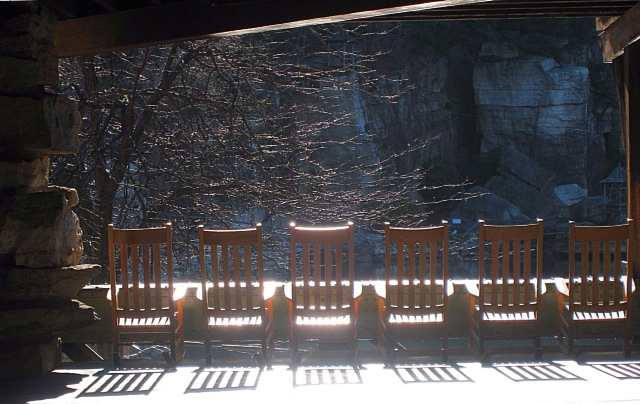The photo captures a serene outdoor-indoor space, likely a rustic restaurant's balcony or patio area. Central to the image are six high-back wooden chairs, all empty and bathed in sunlight, lined up against a stone barrier that runs along the edge of the balcony. These chairs face a stunning, natural vista, which features a tall, leafless tree on the left and a dramatic canyon-like landscape with steep rock formations and the hint of a lake below. The patio itself is sheltered by a structure made of large boulders and rustic wood, giving it a cozy, cottage-like feel. To the far left of the image stands a sturdy stone pillar, while on the right, a subtle detail reveals what seems to be a pagoda or gazebo, adding a touch of architectural interest to the scenic view. The interplay of sunlight and shadow enhances the atmospheric and inviting ambience of the space.